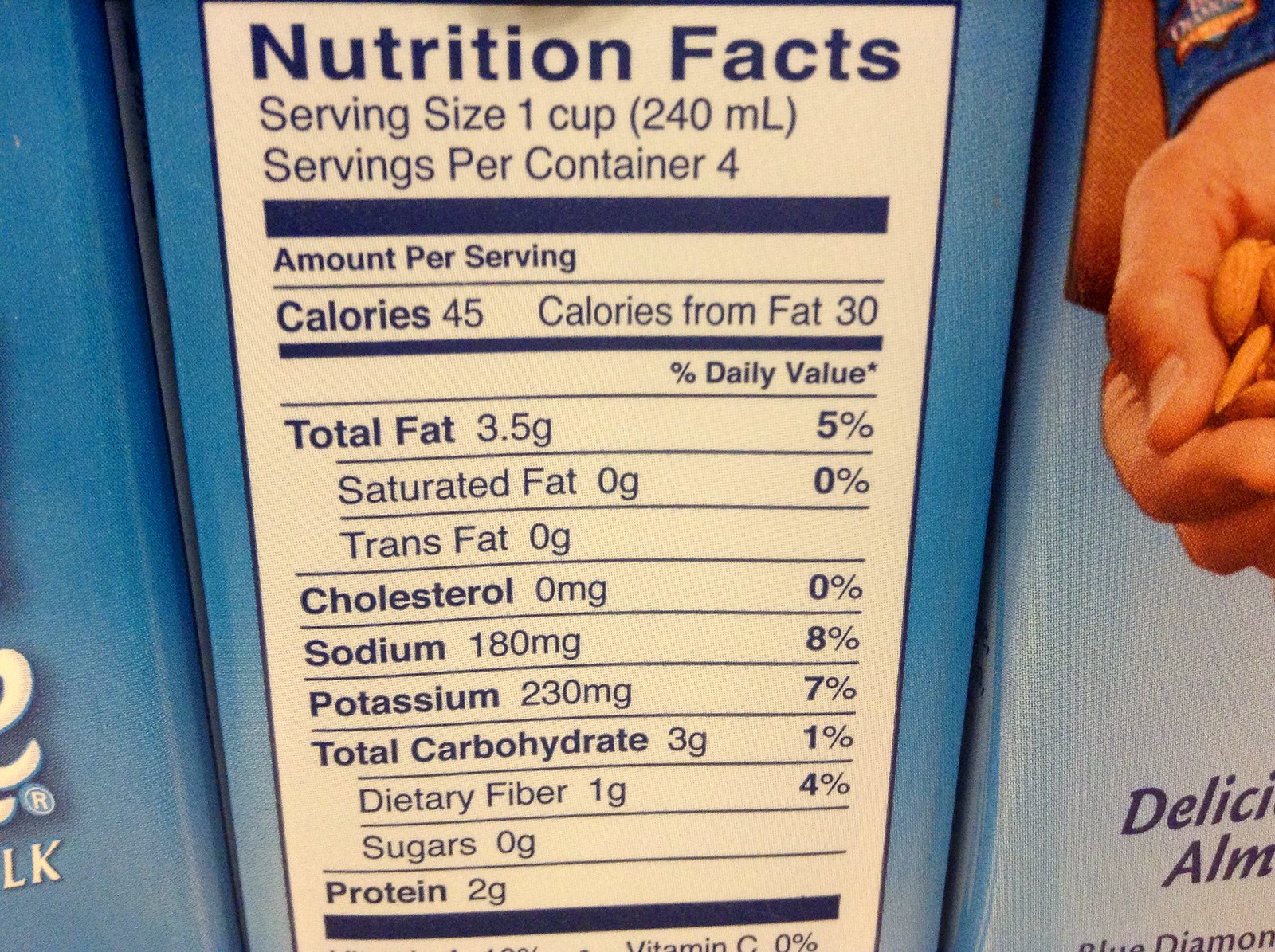This is a detailed caption for a colorful photograph featuring a section of a food box or carton:

The image showcases a portion of a food box or carton, set against a backdrop of similar packages. The primary carton, centrally positioned, sports a blue background and prominently displays a cream or white label with detailed nutritional information printed in dark blue, almost black ink. The label includes standard nutritional metrics such as serving size (one cup, 240 milliliters), servings per container (four), calories, total fat, cholesterol, sodium, potassium, total carbohydrates, dietary fiber, sugars, and proteins. These details are separated by several black bars, and a horizontal black line highlights the bottom section of the table, where a partial red text reads "0%". On the left edge of the central carton, you can glimpse the bordering food box featuring large, white text with just an "E" and "LK" visible. Similarly, on the right, part of another carton appears, distinguished by an image of a person’s hand, colored a vivid orange at the top. The coordinated blue backgrounds of the boxes contribute to the cohesive and visually appealing arrangement.